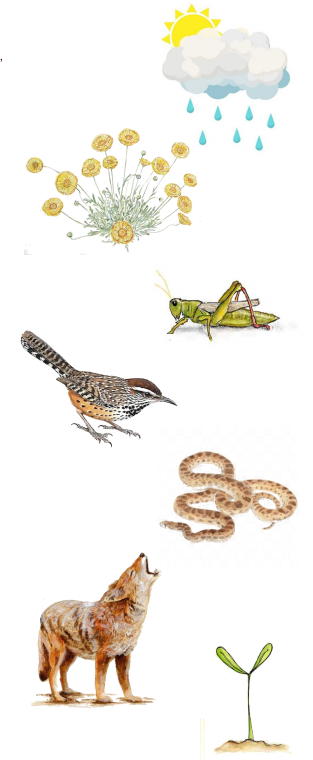The image features a series of detailed, hand-drawn illustrations scattered across a white background, reminiscent of textbook-style artwork, and depicts an array of diverse natural elements. From the top, a white cloud is embedded with blue raindrops falling, partially obscured by a darker blue cloud with the sun peeking out. Beneath this, slightly to the left, is a patch of flowers with skinny green stems and round yellow blooms. Positioned lower and to the right is a light green grasshopper, lying on its stomach, showcasing white wings, yellow antennae, and black eyes. Below the grasshopper and towards the left is a small bird with a brown head and a body adorned with mixed shades of brown, black specks on its underbelly, and a tail featuring black and white stripes. Further down and to the right, a coiled tan rattlesnake with brown spots rests. To the left of the snake, a sable-colored coyote stands howling with its mouth open and eyes closed. At the bottom, toward the right, a delicate plant sprout emerges from a small mound of brown dirt, completing this harmonious illustration of various biological entities.